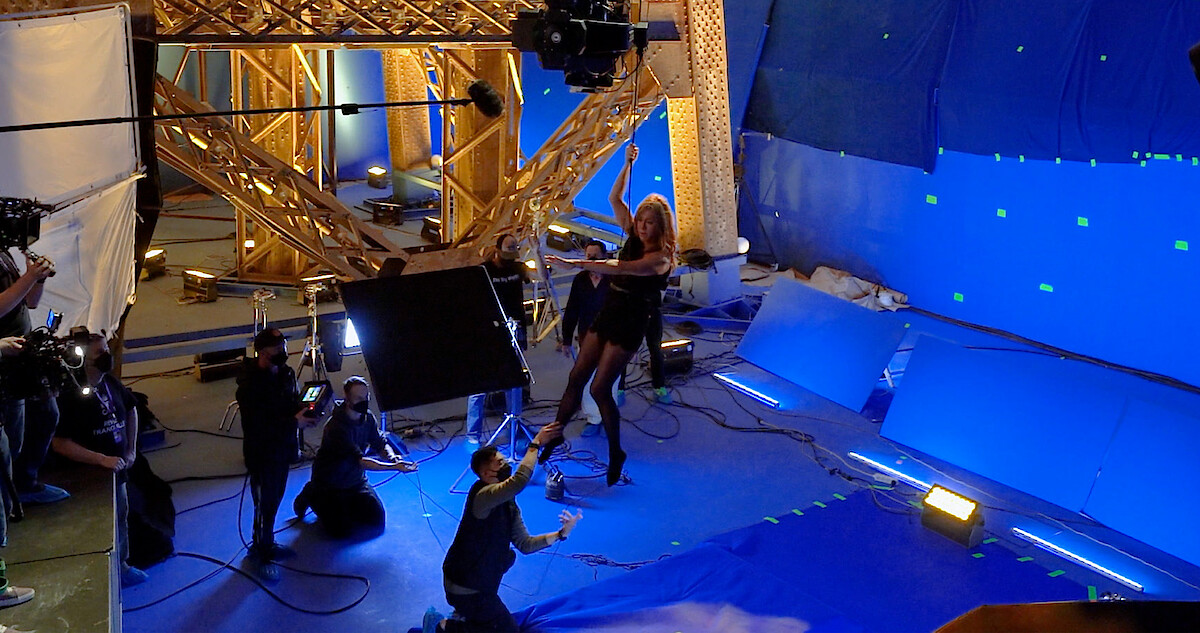In this captivating image, we see a performer being filmed on what appears to be a movie set. The scene is dominated by a royal blue stage that suggests the use of blue-screen technology for CGI effects. The atmosphere is dimly lit, accentuated by structural yellow beams on the left side of the frame. The central focus is a woman with long blonde hair, wearing a tight black mini dress, black pantyhose, and black heels. She is slightly suspended in the air, hanging onto a wire with her right hand while gesturing towards the left with her left hand. Below her, a man squats, holding onto her right ankle – he is wearing a face mask, indicating that this could be during the COVID-19 era.

In the foreground and around the stage, several crew members, also masked, are either kneeling or standing while holding various filming equipment, playing pivotal roles in the production. On the far left, two men are positioned on a raised platform, one holding a camera. Floodlights illuminate the scene from various angles, highlighting the woman and adding to the ambient aesthetic. The intricate setup and the presence of multiple cameras suggest that this is an elaborate filming of a scene, possibly for a film or a high-budget video production.